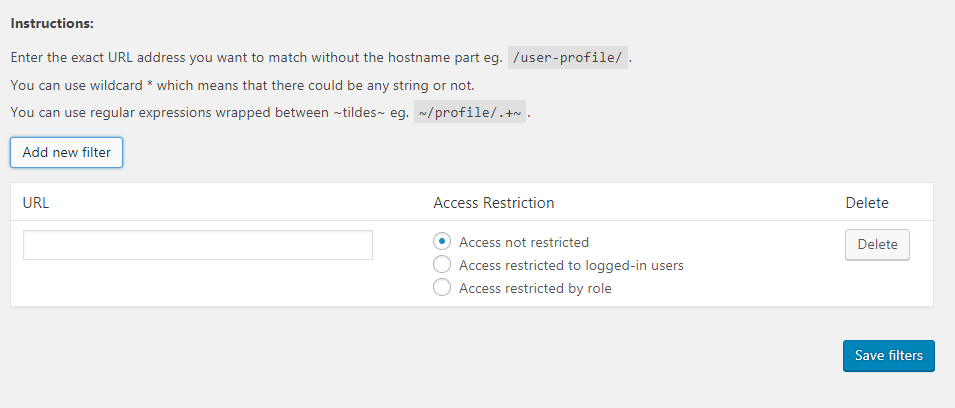The image shows a computer screen displaying a web interface for configuring URL access filters. The background is a gray rectangular box, with the word "Instructions" in black print at the top. Below, it reads: "Enter the exact URL address you want to match without the hostname part". An example is provided in a small rectangle, which says "/user-profile/".

Further instructions explain that wildcards, indicated by an asterisk (*), can be used to match any string or none. It also mentions utilizing regular expressions wrapped between tildes (e.g., `~profile~`), with the example illustrated in another rectangle.

Towards the bottom, there's an "Add Filter" section, displaying an input area labeled "URL". Adjacent to it, there's an access restriction setting with three options: "Access Not Restricted" (selected), "Access Restricted to Logged-in Users", and "Access Restricted by Role". Alongside these options are a "Delete" button and a prominent blue "Save Filters" button.